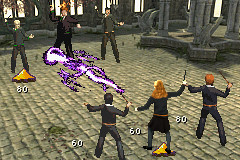The image depicts a detailed in-game screenshot from a Harry Potter-themed video game, featuring a dynamic battle scene set inside a castle. Six characters are engaged in combat on a cobblestone floor with three on each side: Harry Potter, Hermione Granger, and Ron Weasley on the right, and Draco Malfoy with his two cronies on the left. All characters are dressed in black robes, with Hermione distinguished by her black dress and stockings. The characters are wielding their distinctive wands, with Hermione casting a vivid pink or purple energy spell. Numerical indicators display the characters' levels, with Harry, Hermione, and one of Draco's followers at level 60, while Ron and Draco are at level 80. The background features castle architecture, including pillars adorned with decorative gargoyles and large windows. Through the windows, an intense blaze can be seen, hinting at chaos outside.